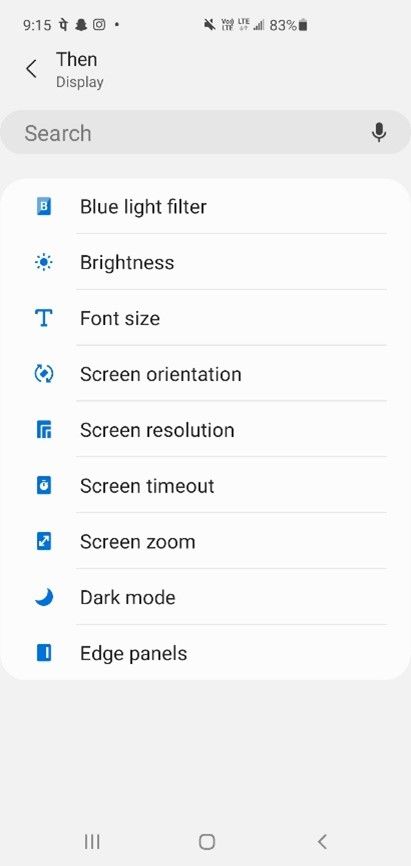A detailed description of the phone screenshot:

The image displays a screenshot of a phone interface taken at 9:15. At the top of the screen, the word "THEN" is prominently displayed. Directly below this, the word "DISPLAY" is visible, accompanying a search box. Inside the search box, the word "SEARCH" is aligned to the left, while a microphone icon, indicating a voice search option, is positioned on the right side of the search box.

Beneath the search box is a list of display-related features, each paired with an icon on the left and descriptive text on the right. The features are listed in the following order:
1. Blue light filter
2. Brightness
3. Font size
4. Screen orientation
5. Screen resolution
6. Screen timeout
7. Screen zoom
8. Dark mode
9. Edge panels

At the bottom of the screen, there are three navigation options:
1. Three horizontal lines (likely representing a menu or multitask view)
2. A circle (commonly indicating the home button)
3. A back arrow (denoting the back button)

This detailed structured layout enables easy navigation and customization of the phone’s display settings.